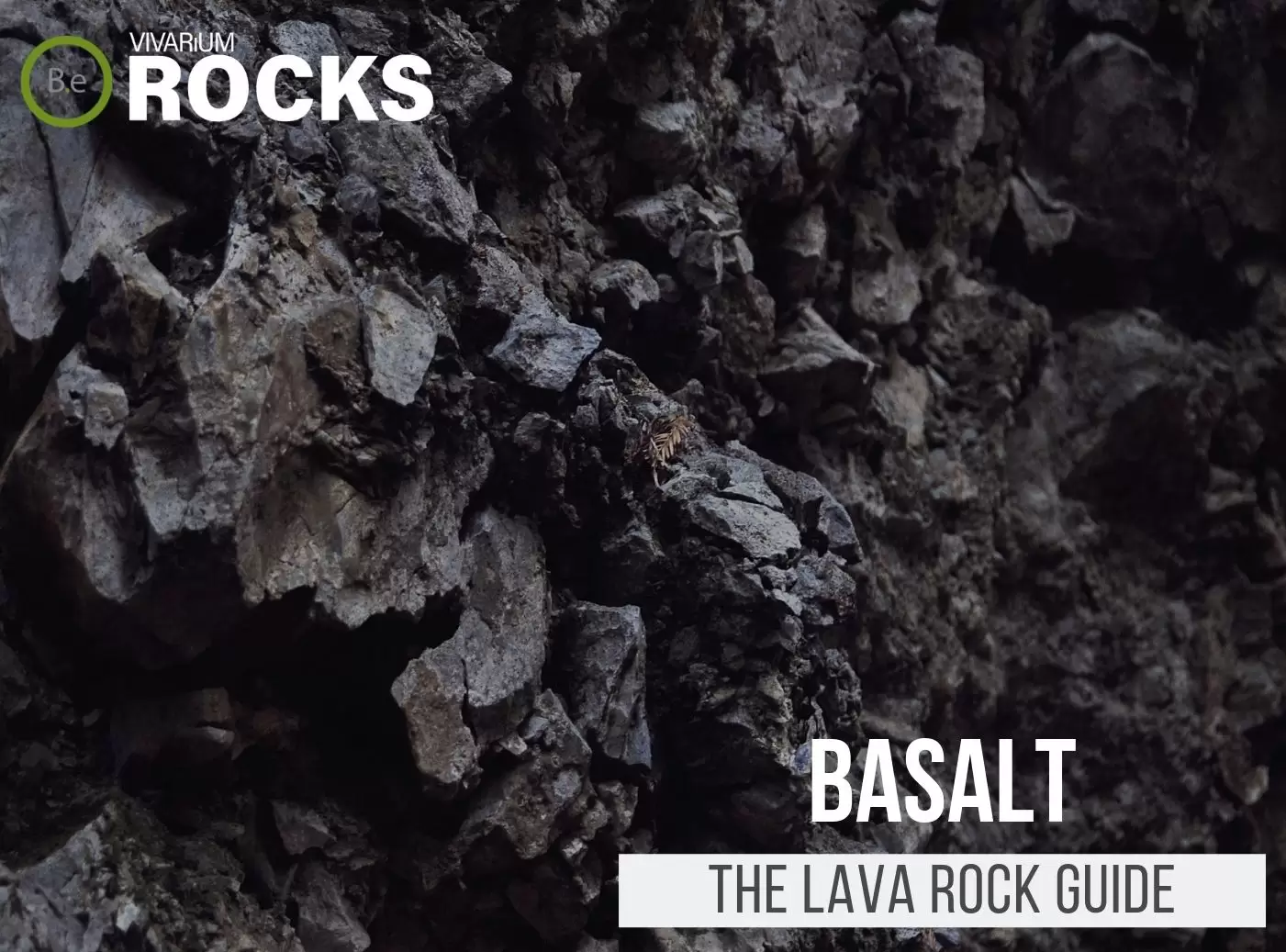This detailed photograph appears to have been taken in or near a volcanic site, showcasing an array of rough, craggy, and jagged basalt rocks that dominate the entire image. The rocks, which display variations of black and dark gray, are most clearly visible on the left side of the image, becoming increasingly blurred towards the bottom right corner. The texture of the rocks is rough and seems to be chipping in some spots, likely due to the volcanic origins.

At the top left, the text "Vivarium Rocks" is prominently displayed in white letters, with smaller gray letters "B.E." encased in a green ring to its left. Near the bottom of the image, "Basalt" is written in bold white letters, and just beneath it, on a light blue rectangular background, the phrase "The Lava Rock Guide" is printed in gray text. A small weed or similar vegetation lies atop one of the rocks, adding a subtle touch of life to the otherwise rocky composition.